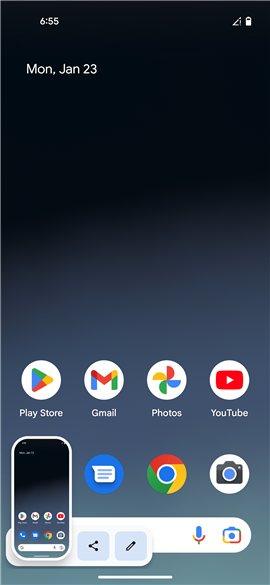The image depicts a smartphone interface characterized by several notable features and distinct coloring elements. At the very top of the screen, the time is displayed in white digits, reading "6:55." Adjacent to it on the right, symbols indicate cellphone reception and battery status with white icons. Immediately below, the date is prominently shown in white text, stating "Monday, January 23rd."

The background of the interface employs a gradient design, transitioning smoothly from a dark black at the top to progressively lighter shades of blue and a subtle hint of green at the very bottom.

Central to the screen are several app icons, arranged in a layout akin to typical smartphone home screens. Among these are the Play Store, represented by a colorful arrow-like symbol, Gmail with its iconic envelope, and Photos marked by a pinwheel design. These icons primarily feature a palette of red, green, yellow, and blue.

To the right, the YouTube icon stands out within a circular border, accompanied by additional icons below it. These include a blue circle with a white speech bubble, likely indicating a messaging app, the Chrome browser icon, and a camera symbol.

At the bottom-left corner of the screen, a screenshot thumbnail can be seen, alongside various editing buttons for further adjustments. Dominating the lower section of the interface, a white search bar extends across the screen, complete with a microphone icon for voice input and a camera icon for visual search capabilities.